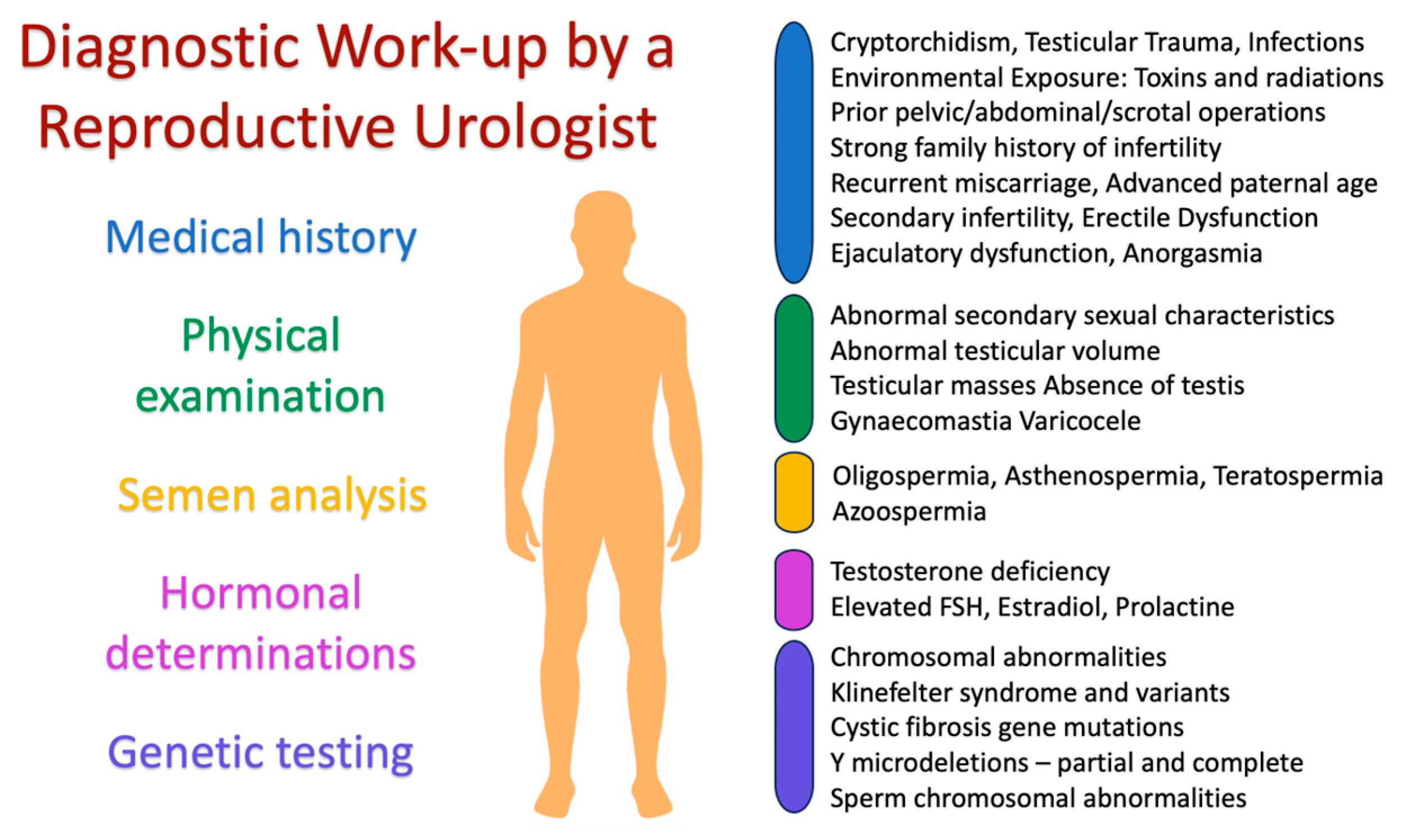The image is an animated chart designed for medical information, specifically a diagnostic workup by a reproductive urologist, as indicated by the red text in the upper left corner. The chart features a yellow-colored silhouette of an adult male in the center. To the left of the silhouette, there is a list of diagnostic categories, each in a different color: Medical History in blue, Physical Examination in green, Semen Analysis in gold, Hormonal Determinations in purple, and Genetic Testing in blue. Each category title is written in black font. On the right side of the image, there are corresponding colored bars, each detailed with paragraphs of black text explaining the diagnostic criteria or procedures for each category. The background of the image is white, providing a clear and uncluttered context for the detailed medical information presented.